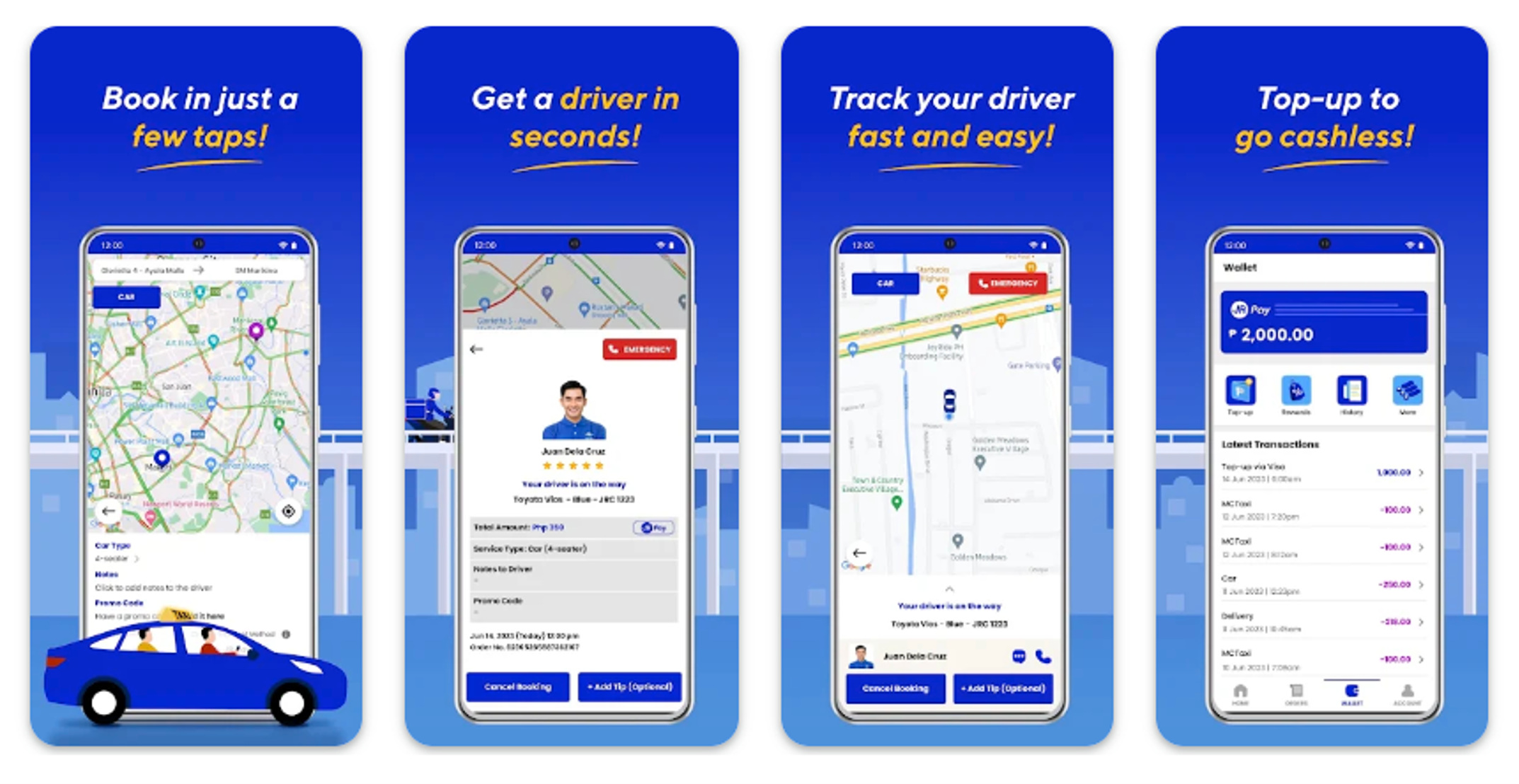This is a detailed and descriptive caption based on the voice-given description:

"A screenshot showcasing an advertisement banner for a mobile application is prominently displayed. The banner features a phone mock-up vividly illustrating the app in use through four distinct sections, each stacked horizontally against a blue background. The first section highlights the feature 'Book in just a few taps,' presenting a phone screen that includes a map interface with a prominent blue button at the top and a blue car icon at the bottom. The second section emphasizes 'Get a driver in seconds,' showing a phone screen with a driver’s profile photo accompanied by a star rating out of five, and two blue buttons located at the bottom of the screen. The third section, labeled 'Track your driver fast and easy,' displays a screen with a blue button at the top and a red button to the right, alongside two additional blue buttons at the bottom. The final section, 'Top up to go cashless,' features a blue banner at the top indicating a balance of $2,000, underscoring the app’s cashless payment option."